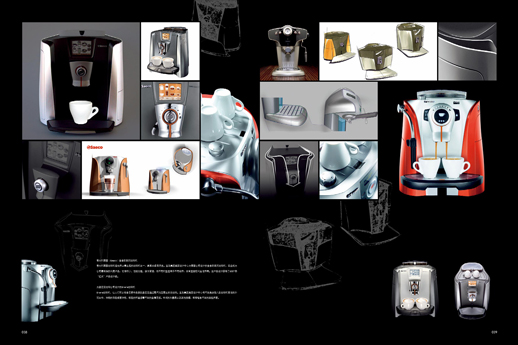The image appears to be an advertisement for a variety of coffee makers, including various models of espresso machines and Keurigs. It features a collage of 16 photographs showcasing different sizes, features, and colors such as black, white, gray, tan, silver, and red. Each coffee maker is displayed individually, likely in stock photos similar to those found on retail websites. These images are arranged on a predominantly black background that includes some illustrative drawings of coffee makers as well as some small, indiscernible white text at the bottom. The collage highlights various functionalities, including machines for single and double cups.